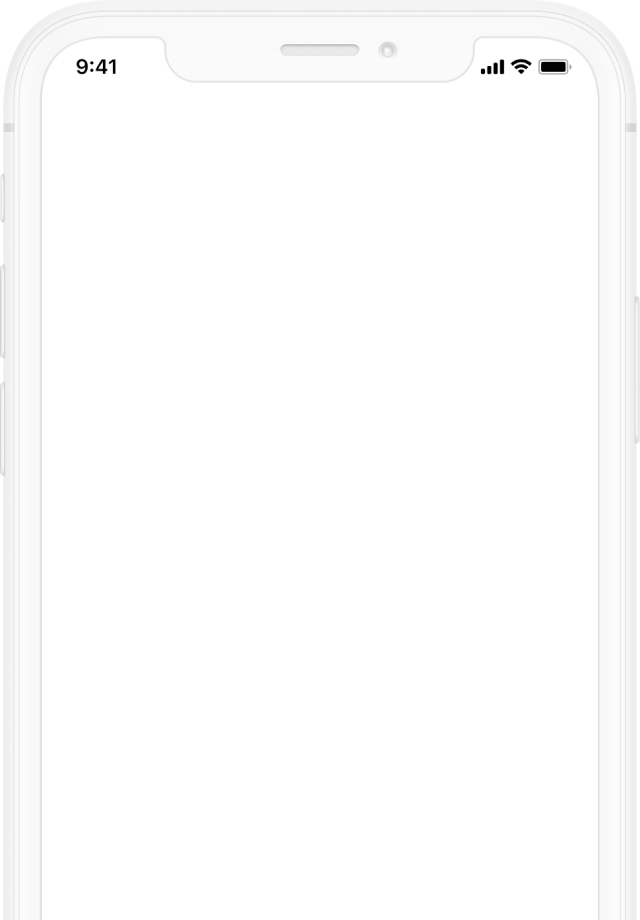A high-resolution image showcases the outline of a sleek, modern smartphone with a minimalistic design. Dominating the screen, the time "9:41" is prominently displayed in black text at the top-left corner. Adjacent to this, at the top-right corner, are fully-loaded icons for signal strength, Wi-Fi, and battery life, all rendered in black. The main screen is stark white, devoid of any icons, images, or other distractions.

Encircling the outer edge of the device, several physical features are discernible. On the left side, positioned higher up, are three distinct buttons—two larger ones and a smaller one situated further up. Additionally, a small pinhole indentation is visible, indicative of a possible microphone or reset feature. The right side houses one large button, opposite another small pinhole, mirroring the left side's design.

At the top of the screen, a small cutout likely accommodates a front-facing camera. Near this cutout, there is a narrow slit, the purpose of which is unclear, but it may function as a speaker grille or another form of sensor. This thoughtful arrangement of elements suggests a focus on both aesthetics and functionality in the smartphone's design.